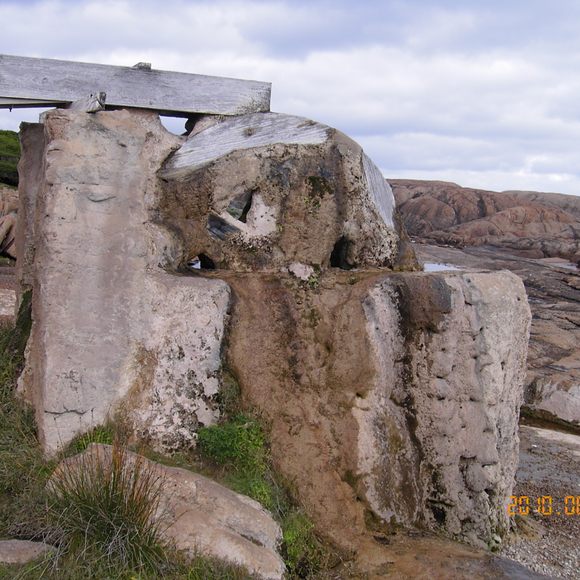This image depicts an outdoor scene featuring a large, weathered rock formation that dominates the frame. The rock itself is primarily brown and gray with patches of white stone and is adorned with moss, giving it a textured appearance. At the top of the rock formation, there is a wooden beam that seems to be part of an old, discolored structure, possibly some historical or abandoned site. 

Surrounding the rock, there are small patches of grass and clusters of flowers, particularly noticeable on the left side of the image. A possible channel or groove suggests that water might flow through this area, though it's currently dry. In the background, white clouds are visible in a hazy, blue sky, contributing to the overall serene and rustic atmosphere. The bottom right of the image features a timestamp reading "2010.08," indicating the date the photograph was taken. Together, these elements evoke a semi-desert landscape, reminiscent of regions like New Mexico, highlighting the natural and rugged beauty of the setting.